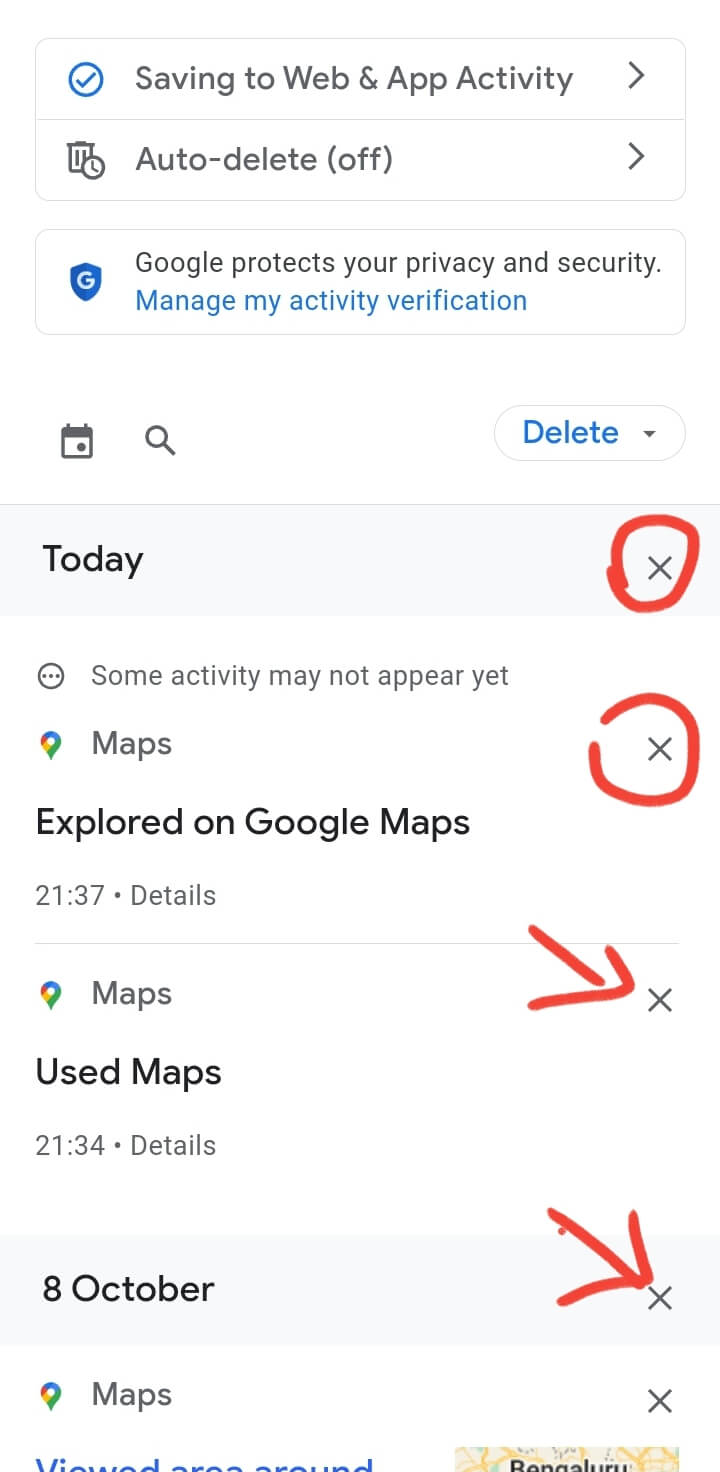The image appears to be a screenshot taken from a phone, likely displaying a Google Activity page. The top of the image features a header with the text "Saving to web & activity." A blue check mark and a blue circle are visible below this header, accompanied by the text "Auto delete off" with a right arrow next to it. Beneath that, the text "Google protects your privacy and security" is displayed, followed by the option "Manage my activity verification."

Further down, there is a calendar icon and a search icon side by side. A delete button with a pull-down menu is also present. The word "Today" has an 'X' on its right side, encircled for emphasis. A note mentions that "Some activities may not appear yet."

The image includes entries related to Google Maps, each entry marked with an 'X' and circled, with red arrows pointing to them. The first entry states "Explore on Google Maps 21:37 detail" followed by a line divider. Another entry reads "Use maps 21:34 details October 8th map," also with an 'X' on the right side and an arrow pointing to it.

All annotations on the screenshot appear to have been hand-drawn using a photo editor, likely for educational purposes. The predominant colors in the image are white, black, blue, gray, and red. Part of the map shown in the screenshot includes shades of yellow and tan, though some sections of the image are cut off.